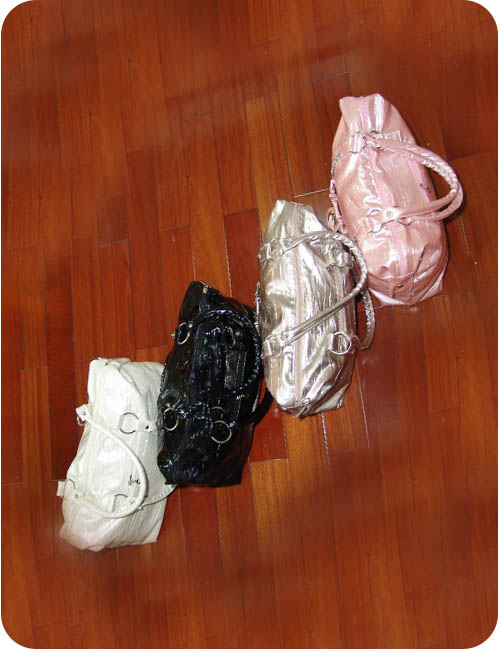The amateur photo is a detailed close-up of four large designer handbags, arranged diagonally from left to right on a wooden floor made up of planks in various shades of brown. Each handbag, which could be made of leather or a thin similar material, features two arm straps held by metal ringlets. The leftmost handbag, positioned in the lower corner of the image, is shiny white with matching white handles and silver rings. To its right and slightly above, the second handbag is a shiny black with black handles and silver rings. Above that is the third handbag, a metallic silver color with matching silvery straps and rings. The fourth handbag, in the upper right section, is a shiny pink with corresponding pink handles and silver rings. The photo has a blurred upper and lower section, with the handbags sharply in focus.